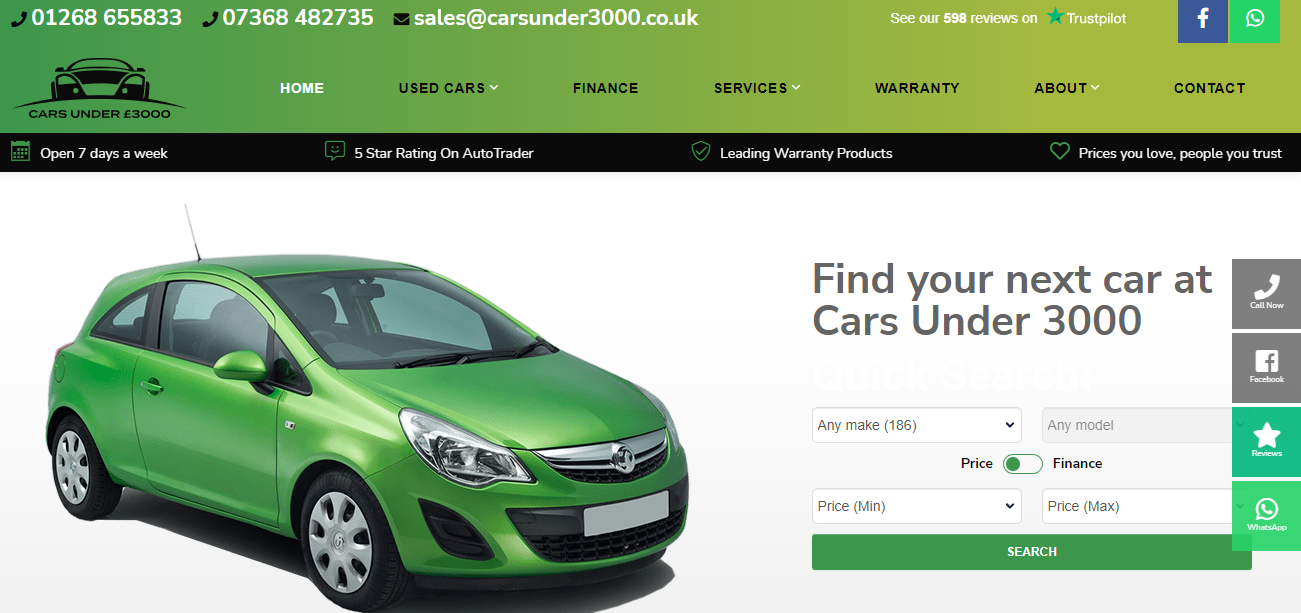In the top section of the image, there is a green box containing various contact options and informational icons. It features a phone icon followed by the number "01268 655833" and another phone icon next to the number "07368 482735". Additionally, there is a letter icon with the email address "sales@carsunder3000.co.uk". Just below this, the text "CR 598 reviews on Trustpilot" is displayed alongside a Facebook icon and a chat icon.

Under these icons, the company navigation bar lists the following sections: "Home," "Used Cars," "Finance," "Services," "Warranty," "About," and "Contact." The image also indicates that the business is open seven days a week and boasts a five-star rating on AutoTrader. They highlight their "leading warranty products" with a unique selling proposition of "prices you love, people you trust."

Further down, a green car image is accompanied by the text "Find your next car at Cars Under £3,000." There's also a dropdown box labeled "Any Make (186)" and a prominently featured green search bar encouraging users to start their vehicle search.